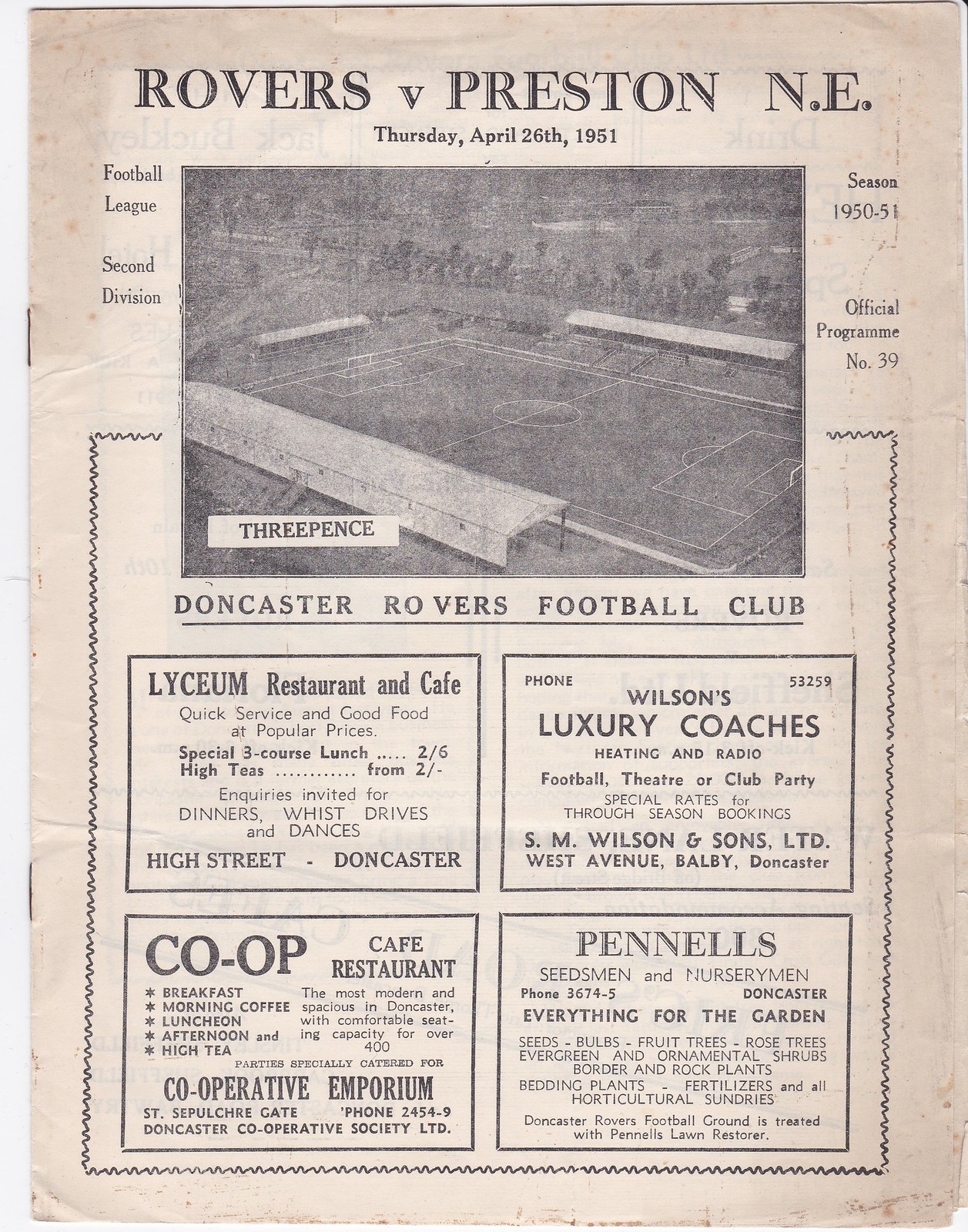This descriptive caption combines the details from each individual's account, focusing on shared and repeated elements:

"This is an aged and slightly worn newspaper clipping featuring an official program for a football match between Rovers and Preston N.E., scheduled for Thursday, April 26, 1951. The event, part of the Football League 2nd Division, Season 1950-51, is listed as Official Program No. 39 and costs 3 pence. The top of the clipping displays a black-and-white overhead photograph of the football field, with visible stands and trees in the background. Below the match details, there are four advertisements: Lyceum Restaurant and Cafe located on High Street in Doncaster, promoting quick service and good food with special 3-course lunches and high teas; Wilson's Luxury Coaches; Pinnell's Seatsmen and Nurserymen offering everything for the garden; and Co-op Cafe-Restaurant of the Doncaster Cooperative Emporium, highlighting its spacious seating for over 400 and services catered for cooperative employees. The page shows signs of age, with staples along the left-hand side, and visible rips, wrinkles, and bent corners, framed by a decorative border around the ads."